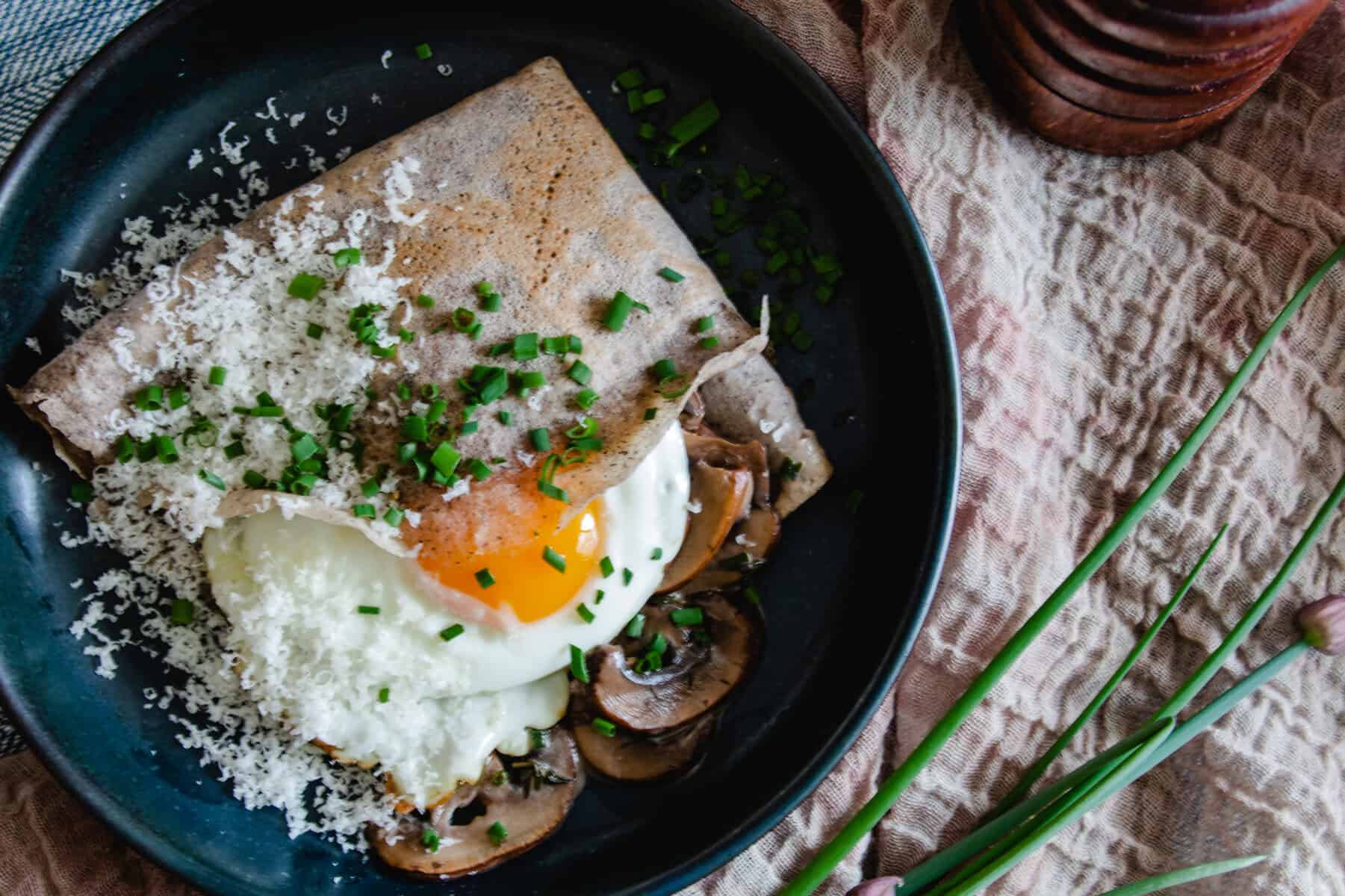A meticulously presented dish rests on a black, Teflon-lined plate, primarily occupying the left side of the frame. The plate sits atop a beige fabric, with a glimpse of blue material peeking from the upper left corner. The main attraction on the plate is a sunny-side-up egg with its vibrant yellow yolk and pristine whites partially covered by a delicate, thin layer of what appears to be phyllo dough or a similar carbohydrate. Surrounding the egg are sautéed mushrooms, adding a rich, earthy tone to the dish. Sprinkled across the ensemble are green herbs, possibly finely chopped chives or spring onions, and a hint of white, crumbly cheese, enhancing both flavor and visual appeal. The right edge of the image reveals a textured, brown crinkly material, on which the plate is set. Just below the midsection on the right and extending towards the bottom, green shoots of a plant inject a touch of nature into the composition. Finally, the upper right corner houses a small, round wooden container, subtly complementing the rustic yet elegant dining presentation.